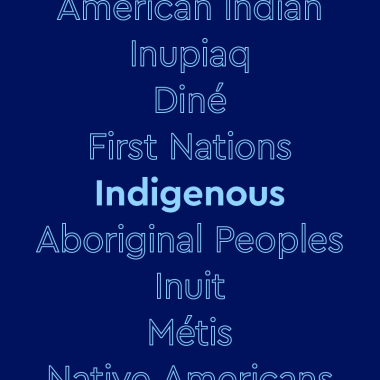The image displays a vertically aligned list of words in the center of a dark navy blue square, which is slightly longer than it is wide. The background is solid dark blue, and the text is primarily outlined in white, making it stand out despite being a similar shade of blue. Starting at the top, the list begins with "American Indian", which is slightly cut off. Following this, the words "Inupiaq" (spelled I-N-U-P-I-A-Q), "Diné" (with an accent over the 'é'), "First Nations", "Aboriginal Peoples", "Inuit", "Métis" (accented 'é'), and "Native Americans" (partially visible at the bottom) appear sequentially down the center. Notably, in the middle of this list, the word "Indigenous" stands out as it is written in a solid light blue color, differing from the outlined style of the other words. There are no additional images, icons, or embellishments, emphasizing the clear and focused presentation of these terms.